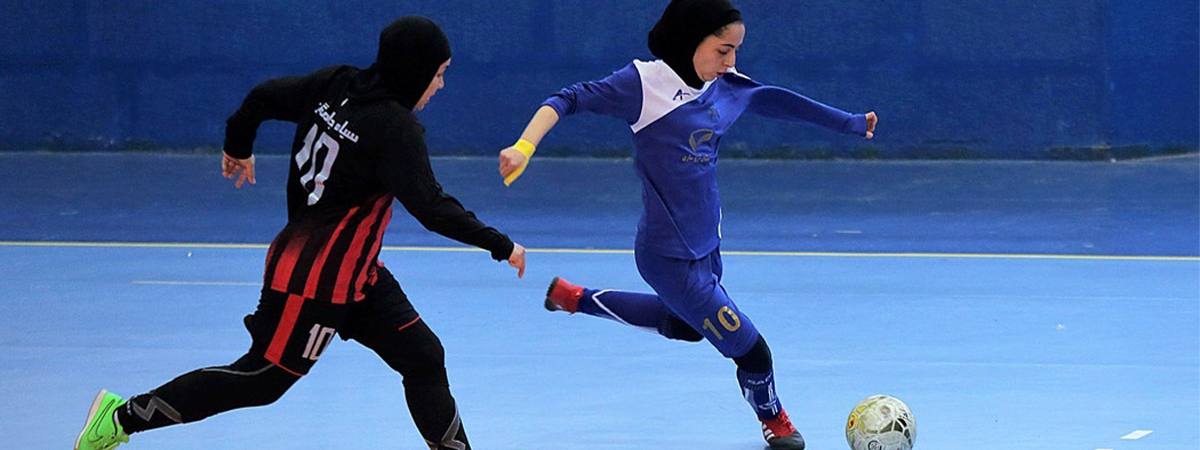In this vibrant action shot, two women are captured mid-game, intensely engaged in an indoor soccer match on a distinctive blue surface. Both athletes are adorned in head coverings, likely indicative of a Muslim country setting. The player poised to kick the white and black soccer ball is clad in a blue uniform accented with white at the top, red shoes, and a yellow bandage that extends from her thumb to her wrist. Her head covering is black. Opposing her is a defender in a black uniform with vertical red stripes, lime green shoes, and a matching black head covering. They are both focused and poised, the defender ready to counter the kick. The blue field, split into lighter and darker shades, and the backdrop wall, frame this moment of intense sporting action, emphasizing the players' dedication and athleticism.